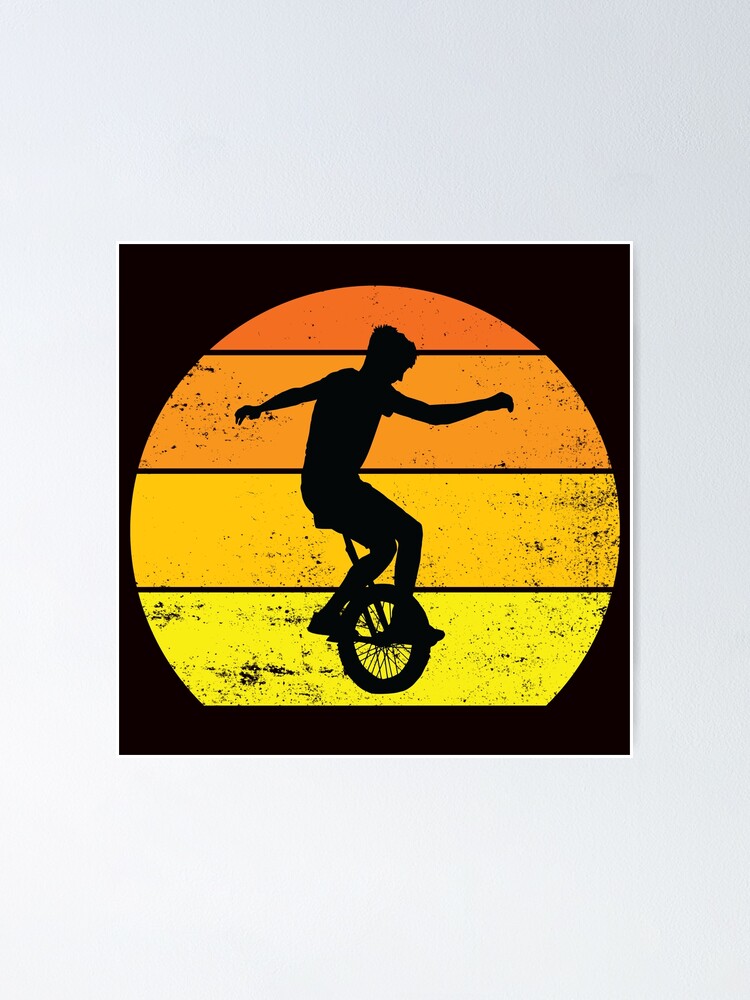The image features a meticulously crafted drawing or painting of a young man silhouetted in black, balancing on a unicycle. He is depicted against a distinctive backdrop that suggests a sunset, with a gradient sun divided into four sections behind him. These sections transition from dark orange at the top to light orange, then to darker yellow, and finally to light yellow at the bottom. The young man, characterized by his short hair and casual attire of shorts and a short-sleeve shirt, has his left arm extended forward and his right arm stretched behind him as if to maintain balance. The entire scene is enclosed within a gray border, set against a black background, creating a striking visual composition.